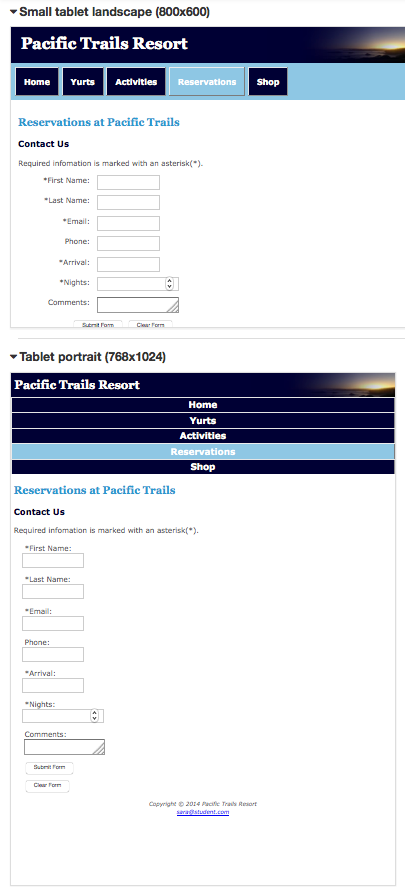Screenshot of a tablet screen, displaying a website interface:

The top section indicates "Small Tablet Landscape" in black font within a white background, followed by dimensions "800 x 600" in parentheses.

Below, a navigational header features a gradient background. Starting from navy blue on the left, it transitions to a warm sunset theme towards the right. Centered within this gradient, the text "Pacific Trails Resort" stands prominently.

Under the header, a menu is laid out within a blue gradient rectangle, featuring several black buttons: "Home," "Yurt," "Activities," and "Shop." A highlighted light blue button, matching the background, indicates the "Reservations" section.

The main content area showcases "Reservations at Pacific Trails" in light baby blue font, followed by a "Contact Us" section. Here, user input fields for contact information and name are provided in the form of interactive chat bubbles.

Finally, the layout concludes with the note "Tablet Portrait 768 x 1024," emphasizing the alternate view format.